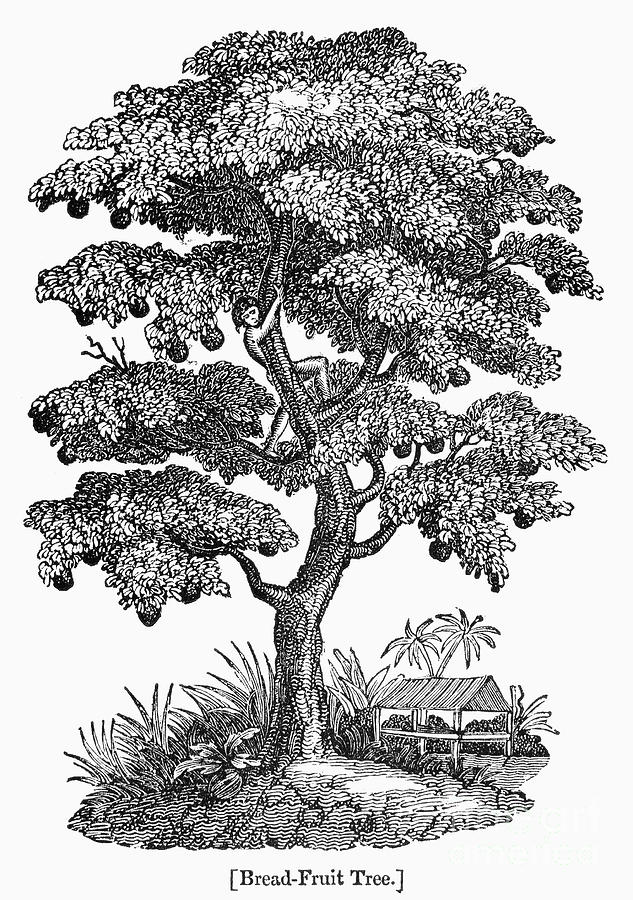This highly detailed, black-and-white illustration appears to be a sketched or possibly a linoleum print image of a breadfruit tree, indicated by the text "breadfruit tree" in square brackets at the bottom of the image. The tree dominates the foreground, emerging from a small, grassy mound adorned with additional plants and rocks at its base. The trunk is sturdy, supporting a large canopy with an abundance of leaves and numerous round fruits, approximately four to five per branch, clustered on its branches.

About halfway up the tree, a young boy, who may be wearing shorts and possibly a hat, is climbing with one foot on the fifth branch and another on the sixth, wrapping his arms around the trunk and peering downward, adding a sense of adventure reminiscent of a scene from "The Jungle Book."

In the background, there are two notable palm trees flanking a dock that extends into the water, covered with a triangular roof. This dock, described as an Asian shed or pergola, adds to the impression that the scene is set in a lush, perhaps tropical locale. The entire composition feels like a carefully crafted illustration from an older children's storybook, rich in detail and shaded entirely in black and white.